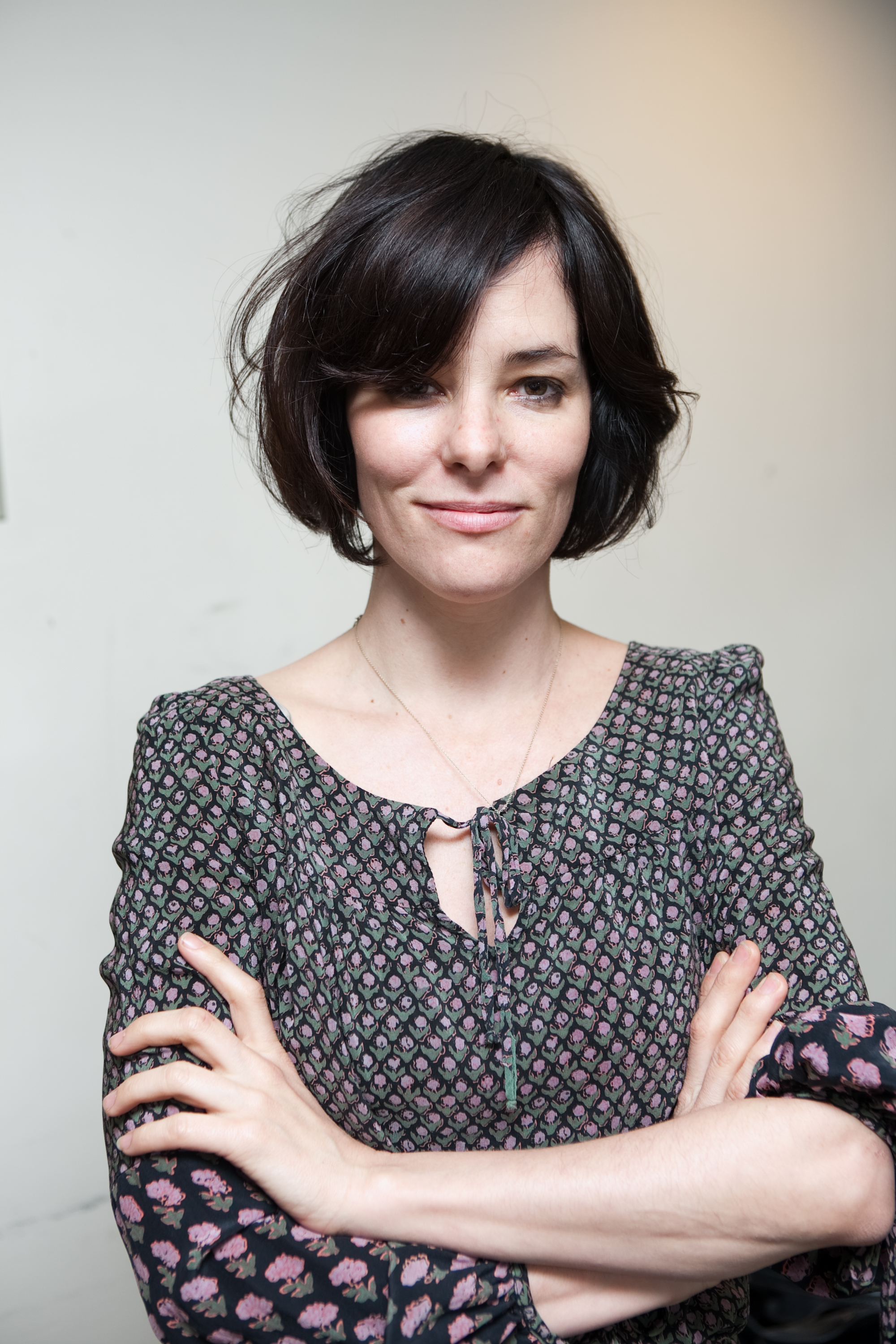In this vertical, rectangular photograph, a woman is standing with her arms crossed, appearing from the waist up. She is a Caucasian woman, likely in her thirties, with short, dark hair styled with a half-bang that covers her right eye, offering a full view of her left eye. She wears makeup and earrings, and a thin gold chain necklace around her neck. Her expression shows a closed-mouth smile that accentuates her dimples.

Her outfit is a long-sleeved dress or blouse, primarily black with small purple polka dots or possibly tiny flowers. The pattern changes from her elbows to her wrists, where larger purple flowers appear. The top features a tie just below the center of her chest, creating a keyhole view of her skin. The background is predominantly whitish-gray with a hint of yellow hue in the upper right-hand corner, giving the setting a neutral and somewhat stark appearance.